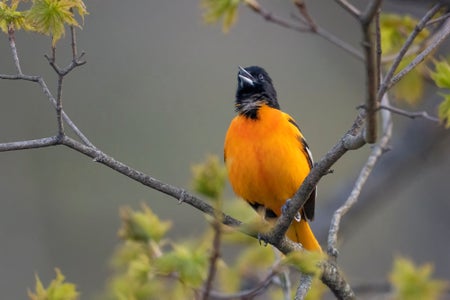In this outdoor photograph, the background is intentionally blurry, appearing as a grayish mush that could be the sky or distant trees. The foreground features a small tree with thin, light grayish-brown branches adorned with star-shaped, yellow-green leaves that are scattered throughout. Positioned almost centrally in the image is a small bird perched on one of the branches. The bird, with its bright orange chest and belly, has a black head, beak, and markings on the edges of its feathers and around its neck. Its dark gray talons grip the branch firmly. Though only the front and side of the bird are visible, it appears to be looking up, slightly to the left, with its beak open, possibly tweeting. The underparts of its wings visible in the photograph are also black, adding to the contrasting colors of this charming avian subject.